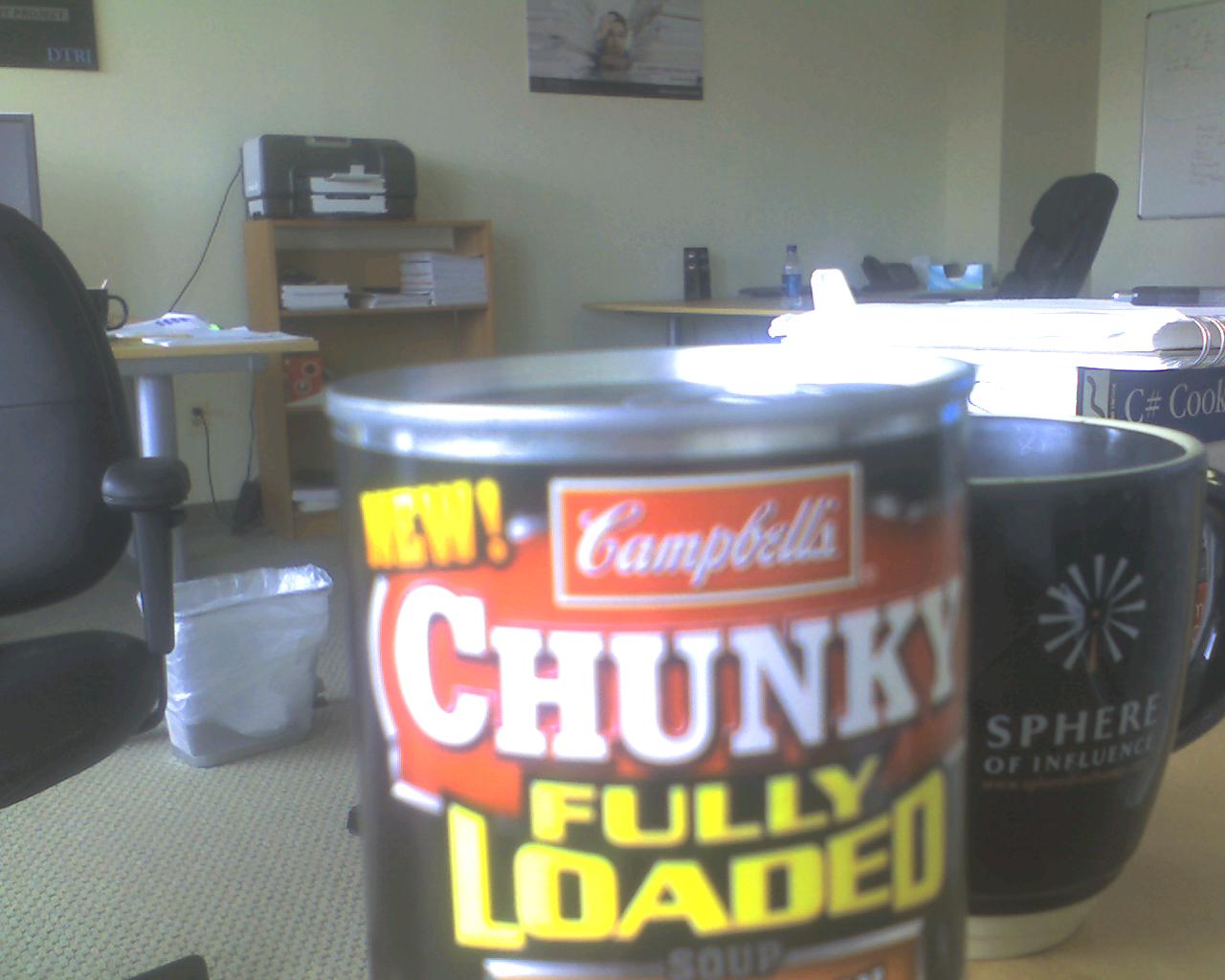In this somewhat blurry photograph, the most prominent feature is a can of Campbell's Chunky Fully Loaded Soup, with only the top portion down to the "Fully Loaded" label visible. The iconic Campbell's logo is shown in bold white letters on a red background, while "Chunky" is displayed similarly and "Fully Loaded" stands out with yellow letters on a black background. This can rests in the foreground on what seems to be an oak-colored surface, possibly a desk or kitchen counter.

Directly to the right of the can is a black coffee mug featuring a white icon resembling a Ferris wheel or flower and the words "Sphere of Influence" written in white. 

In the background, there is a glimpse of a standard office environment. A black desk chair is visible along with a bookcase filled with stacks of paper. Further into the room, you can see a printer along the wall, a wastebasket on the beige carpet, and a whiteboard in the top right corner. There are also posters and additional desks, completing this typical office setting.